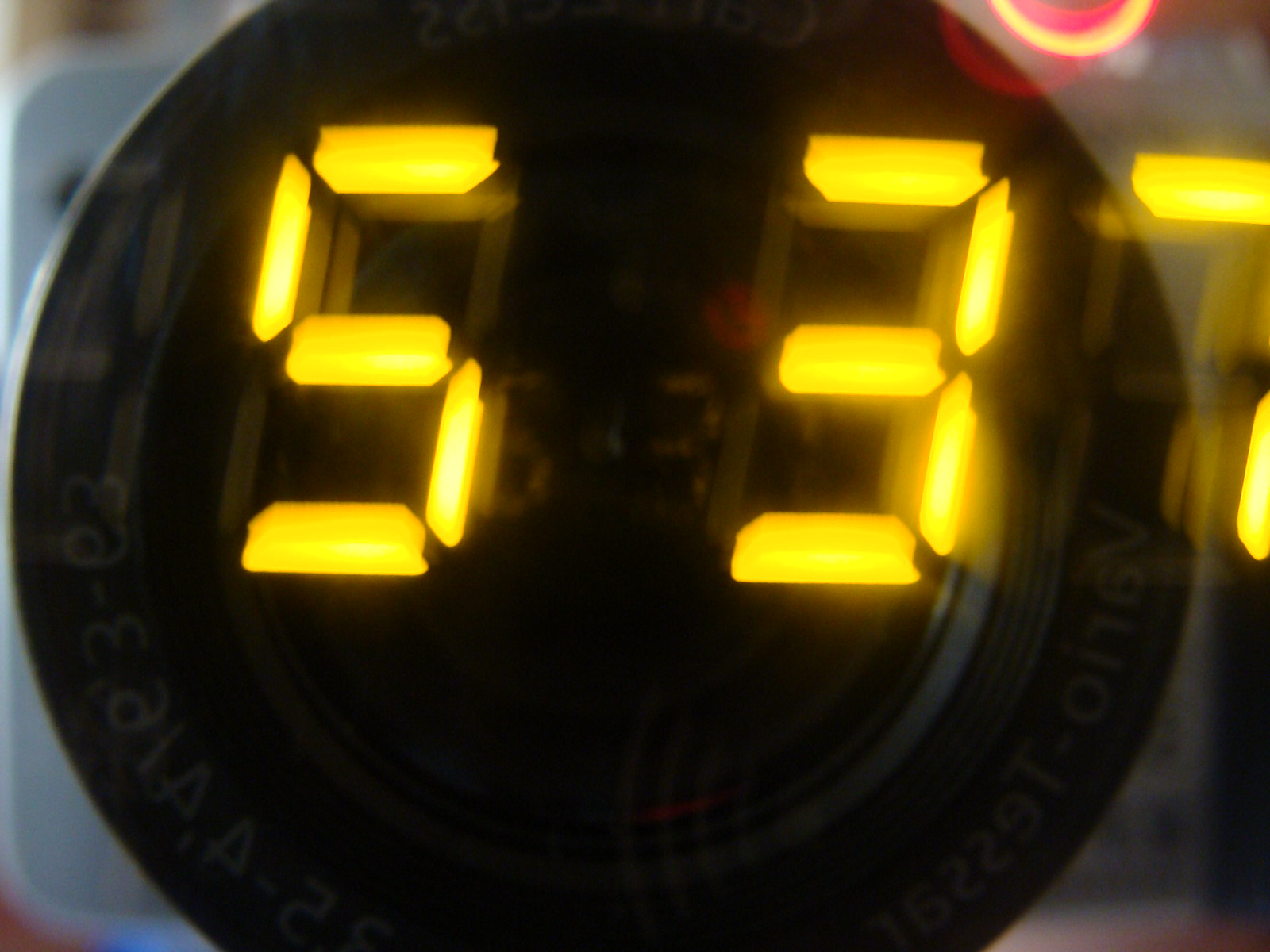The image is an extreme close-up of bright yellowish-orange neon numbers "537" on what appears to be a digital clock or timer. Set against a black plastic cover and black background, the image shows a circular black area resembling a camera lens with a mirrored reflection of the "537" numbers within it. The photograph is slightly blurry and includes a faint reddish light at the top right. Additionally, the outline of another number, potentially part of the LED display, is barely visible beneath the "537". The face of the camera capturing the photo is also reflected, and there's an obscured red circle above the main numbers.